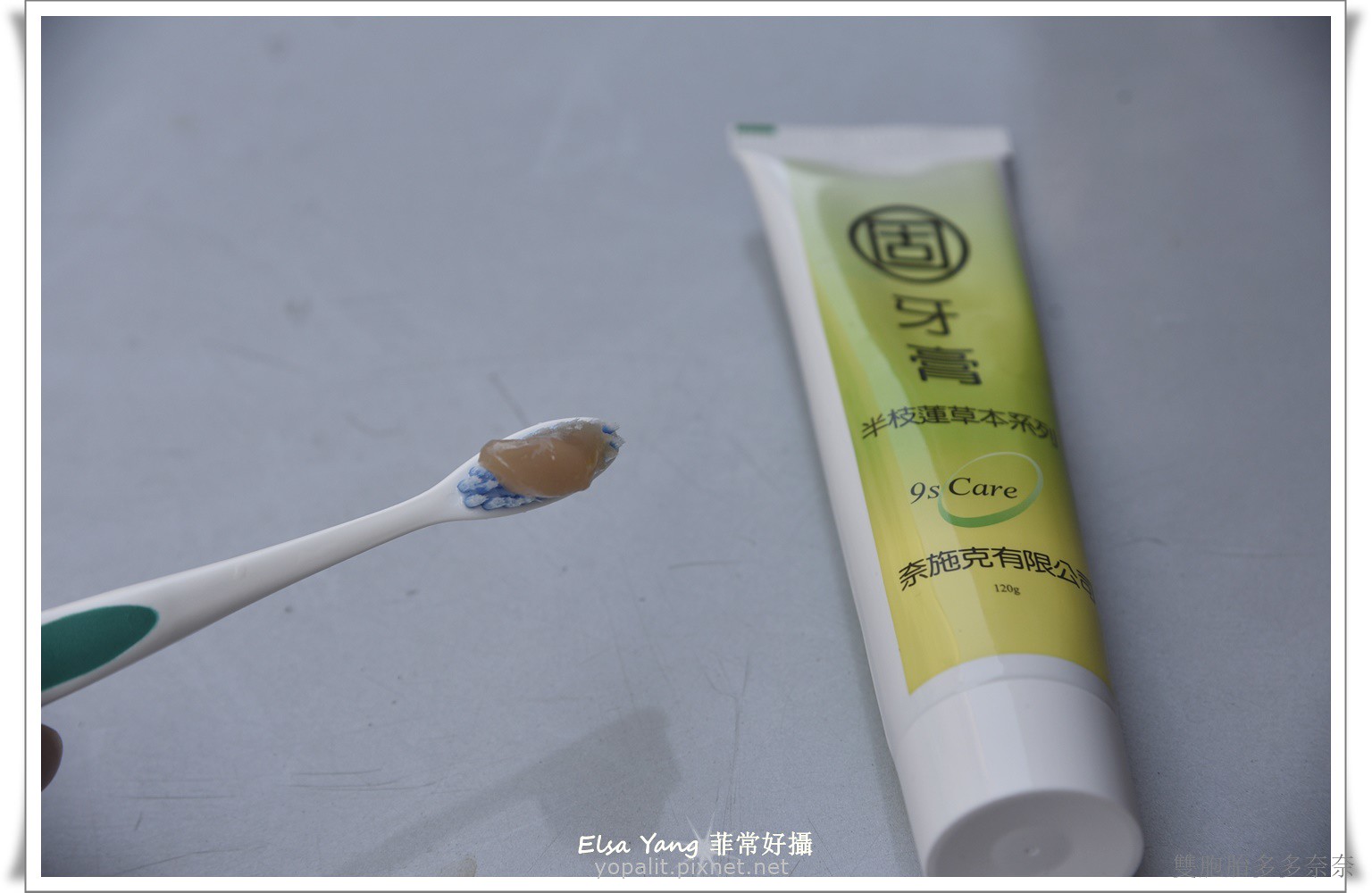This landscape photo showcases a white toothbrush prominently held diagonally from the bottom left to the center. The toothbrush displays an oval dark green accent in the middle and has bristles that are a mix of white and blue, currently smeared with a brown peach-colored toothpaste. In the bottom left corner, the tip of a finger, likely from the hand holding the toothbrush, is visible. The image also includes a white tube of toothpaste positioned to the right of the toothbrush, featuring a lime green and yellow front label with Japanese or Chinese characters and the English phrase "9th Care." The white tube is capped with a circular lid and lies against a gray-white countertop background that appears scratched and dingy. Additionally, at the bottom of the image, in white text, are the names "Elsa Yang" and "yoplay.picsnet.net," accompanied by more foreign characters.